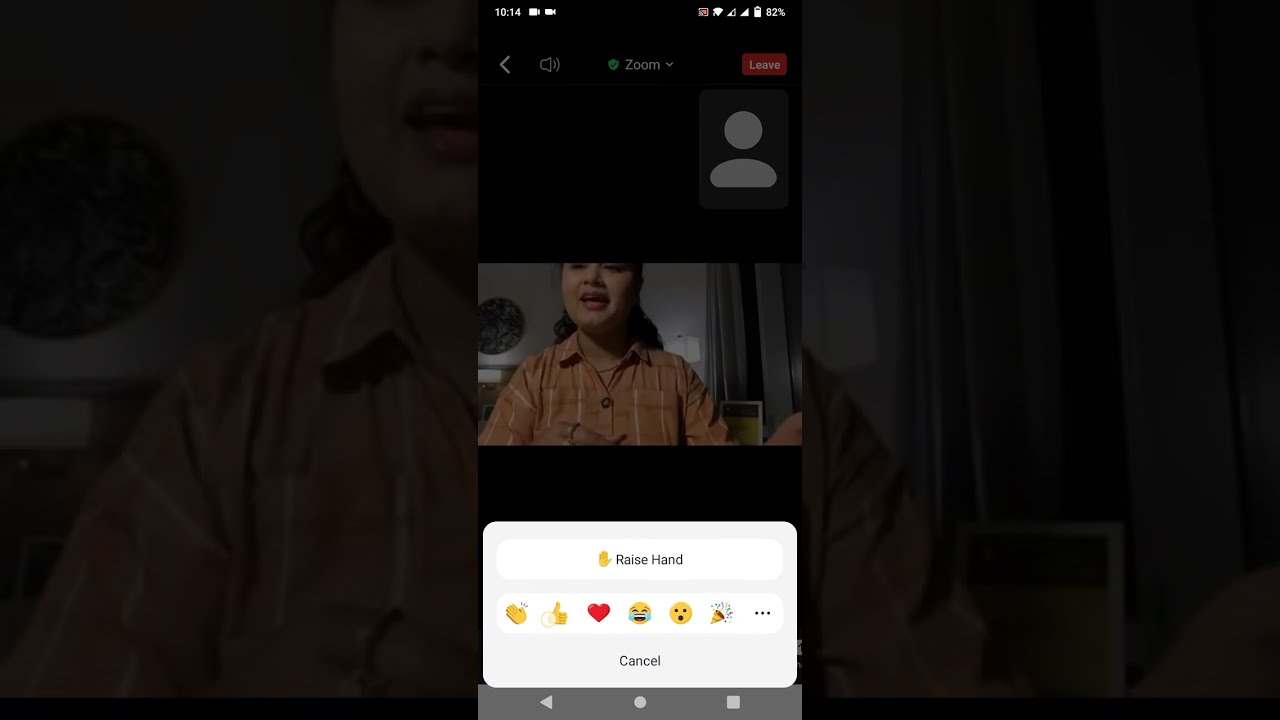In the image, a woman in her twenties, possibly of Indian or Asian descent, is participating in a Zoom call on her smartphone. She is wearing a brown collared shirt with pockets and a necklace, and her medium to long hair frames her smiling face as she engages with the camera. The dark background suggests she might be in a bedroom, evidenced by a visible round picture or globe on the wall and a lamp sitting on a table. The smartphone screen displays the time as 10:14, the battery at 82%, and a Wi-Fi connection. At the top of the image, icons denote camera and data usage. The Zoom interface is clearly visible, featuring a red "leave" button, and a white bar at the bottom with emoji reactions such as "raise hand", "clapping", "thumbs up", "heart", "laughing", and a "celebration" emoji, indicating the interactive elements of the call.